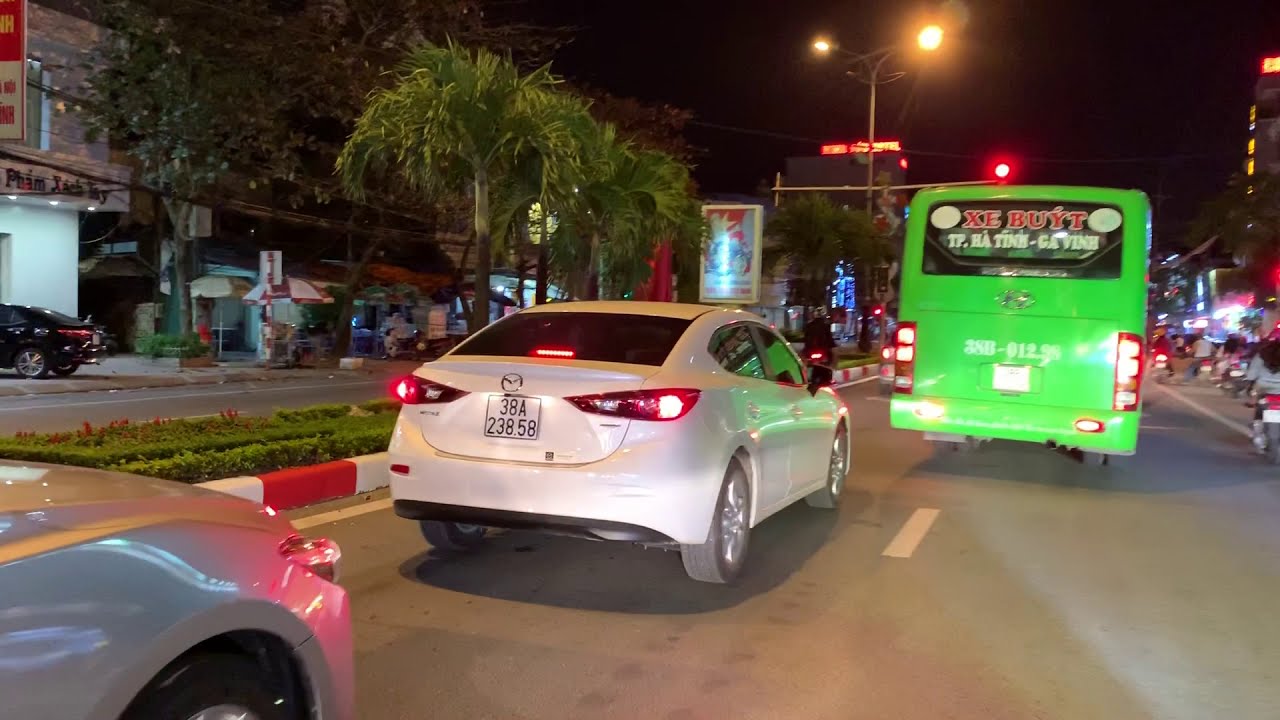This nighttime outdoor photograph captures a busy road scene illuminated by streetlights. Prominently, a bright green bus with red text on its rear is visible, followed closely by a white car with glowing red taillights and another vehicle, of which only the front portion is seen. The road features a dotted white line and is bordered by a green grass median with various plants. On either side of the road are buildings and houses, some of which appear to be restaurants with umbrellas or awnings, though their colors are indiscernible due to the distance. People are visible along the sidewalk, and parked cars can be seen to the left. The sky overhead is dark, accentuating the artificial light that illuminates the scene. Overall, the colors in the image include lime green, red, white, gray, dark green, black, and various shades of blue, red, green, brown, and silver, emphasizing the vibrant and detailed urban setting.